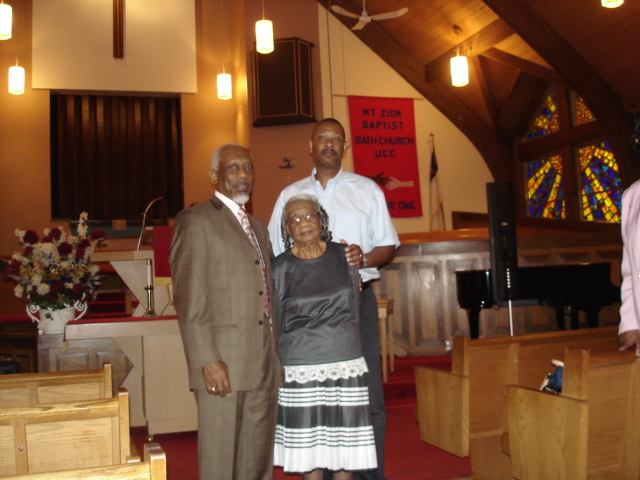This image captures a poignant moment inside the Mount Zion Baptist Bath Church, UCC, featuring three African-American individuals standing centrally within the church's serene interior. The structure of the church includes wooden pews, visible on both sides with three on the left and two on the right. The church's architecture is accentuated by a vaulted wooden ceiling and a red carpeted floor, adding to the warmth of the setting. The background features an inscription reading "Mount Zion Baptist Bath Church, UCC," along with flowers in a vase and a stained-glass window to the right. The lighting includes bulbs hanging from the ceiling, casting a gentle glow throughout the space.

The central figures in this image consist of an elderly man, an elderly woman, and a younger man. The man on the left, who appears to be around 60 or 70 years old, has grey hair and a white beard. He is dressed in a gray suit with a white shirt and tie, his right arm resting at his side. To his right stands an elderly woman, approximately 70 years old, wearing a dark gray dress with white stripes at the bottom, which may appear as a pleated skirt. She also seems to have a jacket on, though her arms are not clearly visible. Behind her and slightly to the right is a younger man, perhaps in his 30s, with short dark hair, dressed in a white short-sleeved shirt and grey or blue dress pants. His left hand rests gently on the elderly woman's shoulder.

The harmonious mixture of colors in the image, ranging from shades of brown in the pews and ceiling trusses to the woman's attire and the red carpet, contributes to a cohesive and warm visual ambiance, capturing a moment of unity within this spiritual and serene church setting.